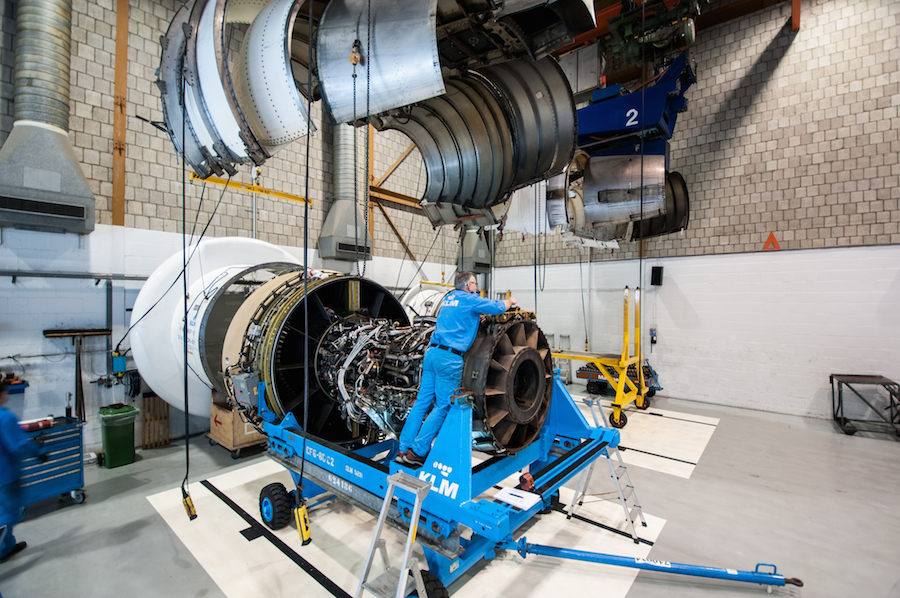In a horizontally aligned rectangular image taken inside a busy workshop or manufacturing facility, a man in a blue shirt and jeans is painstakingly working on a large, complex cylindrical machine that seems to be part of an airplane engine. The machine bristles with intricate wires, pipes, gears, and other mechanical parts, and is mounted on a robust blue metal trailer-like apparatus with a long handle. This apparatus, equipped with small black wheels and blue rims, is designed to transport heavy machinery and bears the white print "KLM." 

In the background, the tall stoned wall is painted white up to about six feet, above which it transitions into brown bricks. There's another man, blurry and in motion, on the lower left side of the image, seemingly walking towards the focus of the scene. To the left, a blue tool cabinet and a green wastebasket can be seen, while a variety of colored pipes and details such as a gray, yellow, and blue pipe, and a blue item marked with the number "2" add to the cluttered, industrious atmosphere. Above the central machine, metal frames and possibly other metal components hang from the ceiling, suggesting ongoing construction or assembly tasks.